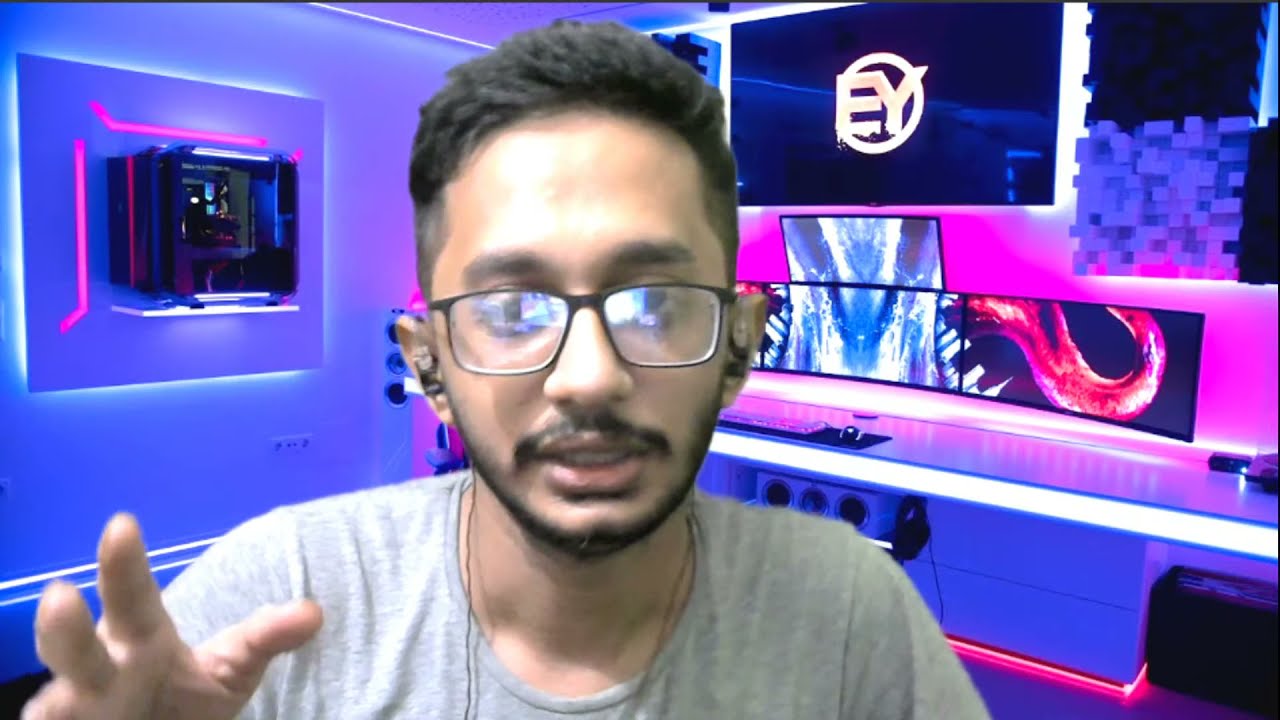In this striking and vivid image, a man of Middle Eastern or Southeast Asian descent gazes directly into the camera, his intense expression framed by black, rectangular reading glasses that catch a distinctive glare from the surrounding lights. His neatly trimmed short black hair with shaved sides, a mustache, and a slight beard create a polished yet approachable appearance. He is engaged, possibly speaking or making a point, as his right hand is partially raised towards the camera. Adorning his ears are black earbuds, and around his neck dangles a thin black cord, perhaps a necklace or chain, partially obscured. 

The man wears a simple gray t-shirt, contrasting the vibrant background which is illuminated with striking neon hues of pink, blue, and purple. Behind him, multiple monitors dominate the scene, contributing to a futuristic ambiance. Notably, one monitor features a logo with a capital 'E' and 'Y' encircled in white, with the monitor itself framed in white. Below this, additional screens with marble-like backgrounds variously light up the space. The setting appears to be a high-tech indoor environment, possibly a gaming or streaming setup, accentuated by the colorful lighting and plethora of screens.